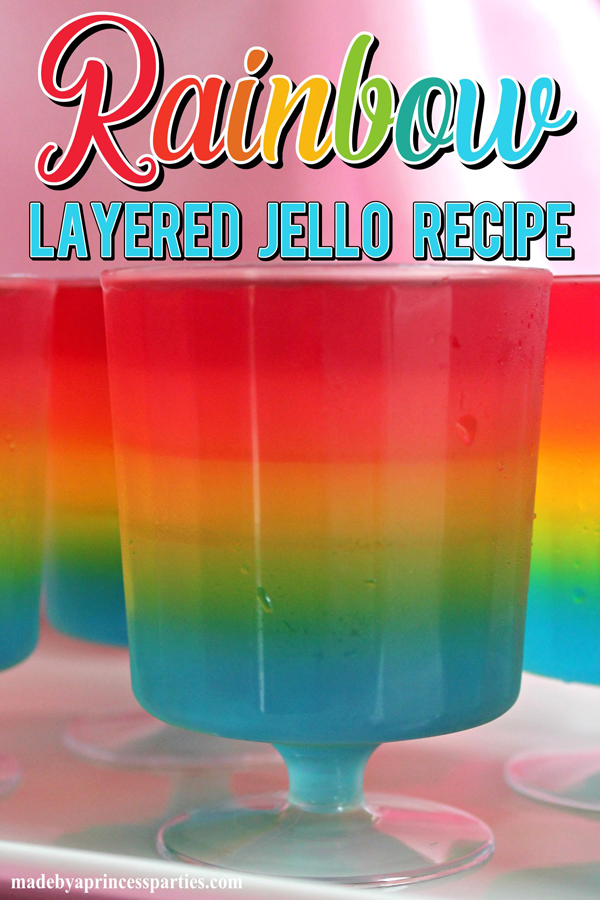This is a vertically-oriented photograph, similar to a portrait layout, featuring a promotional image for a 'Rainbow Layered Jello Recipe.' At the top of the image, the text 'Rainbow Layered Jello Recipe' appears, with each letter in rainbow colors—red, orange, yellow, green, teal, and blue—matching the vibrant hues of the Jell-O layers. Below this, in smaller teal text, the caption continues to describe the recipe. Additionally, the bottom left corner of the image has a watermark reading 'Made by PrincessParties.com.'

The main focus is several tall, narrow cups, resembling potted plant containers with flared bases and thin stems. There are four cups in the frame, with one in the foreground and three in the background (two on the left and one on the right). Each cup is filled with multi-tiered Jello, starting from blue at the bottom, transitioning through green, yellow, and orange, up to red at the top, creating a gradient that mirrors the rainbow. These cups are arranged on a white plastic tray, emphasizing their colorful contents.